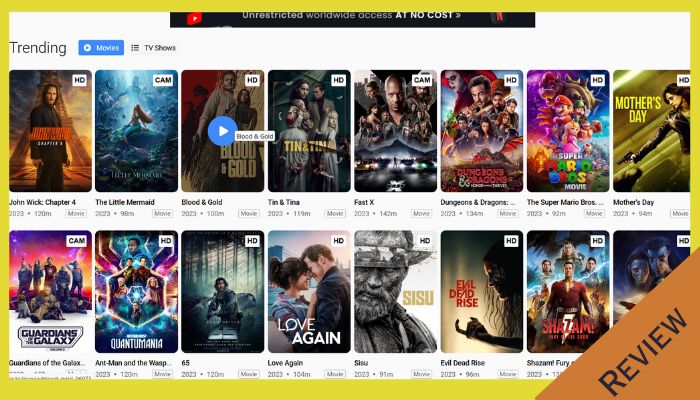This image, captured from a computer screen, prominently features a dark rectangular banner at the top center that reads "Unrestricted Worldwide Access at No Cost." On the left-hand side, the word "Trending" appears, followed by a rectangular button labeled "Movies" with an arrow inside it. Beneath this, there are icons resembling clickable bars, and the label "TV Shows."

The main portion of the screen showcases a grid of 16 TV show or movie thumbnails arranged in two rows of eight. Surrounding the entire image is a yellow border line. In the bottom right corner, there is a small orange tab marked "Review."

The thumbnails displayed in the top row, from left to right, include:
1. John Wick: Chapter 4
2. The Little Mermaid
3. Blood and Gold
4. Tin and Tina
5. Fast X
6. Dungeons and Dragons
7. The Super Mario Bros.
8. Mother’s Day

In the bottom row, the thumbnails are:
1. Guardians of the Galaxy
2. Quantumania
3. 65
4. Love Again
5. Sisu
6. Evil Dead
7. Shazam
8. An incomplete title, cut off at the edge of the screen

The composition and details of this image suggest a streaming platform interface, highlighting popular content and featuring a navigational layout designed for user engagement.